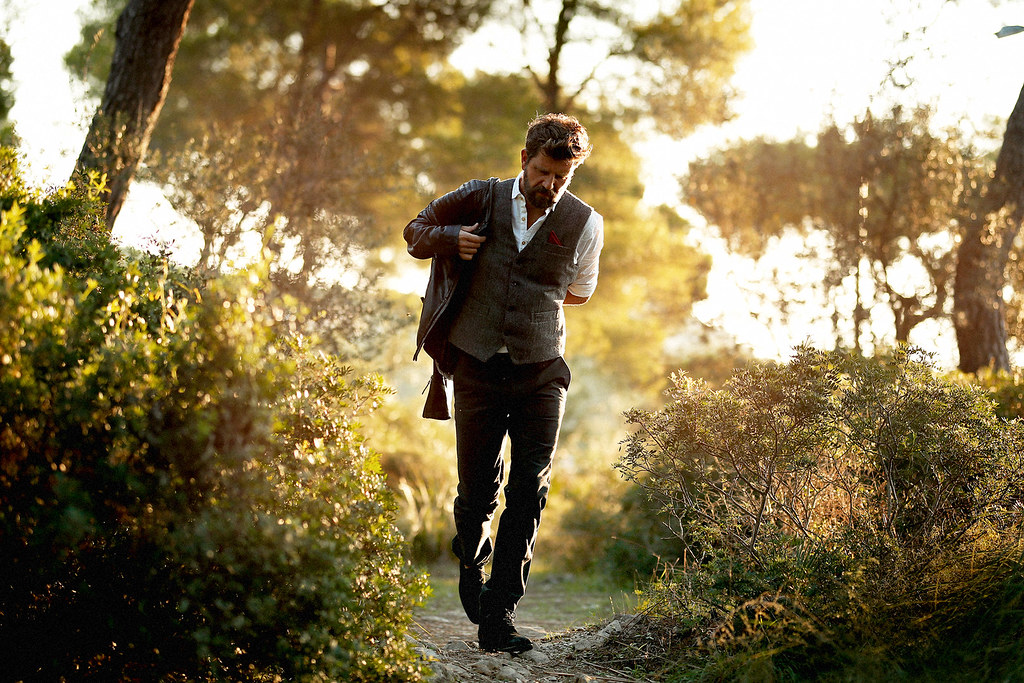In the photograph, a middle-aged Caucasian man with short brown hair and a beard is captured walking down a dirt and rock-strewn trail through a forested area. He is donning a gray vest over a white shirt with rolled-up sleeves, and he seems to be in the process of putting on a maroon leather jacket. His right arm is already through the sleeve, while his left arm is reaching behind him to complete the action. He wears dark pants and black shoes. The sunlight illuminates him from the right side, creating a reflection on his pants. Surrounding him are lush, bushy green and orangish trees, with a tree trunk visible in the left background. The sky above is overcast, giving a white backdrop to the scene.